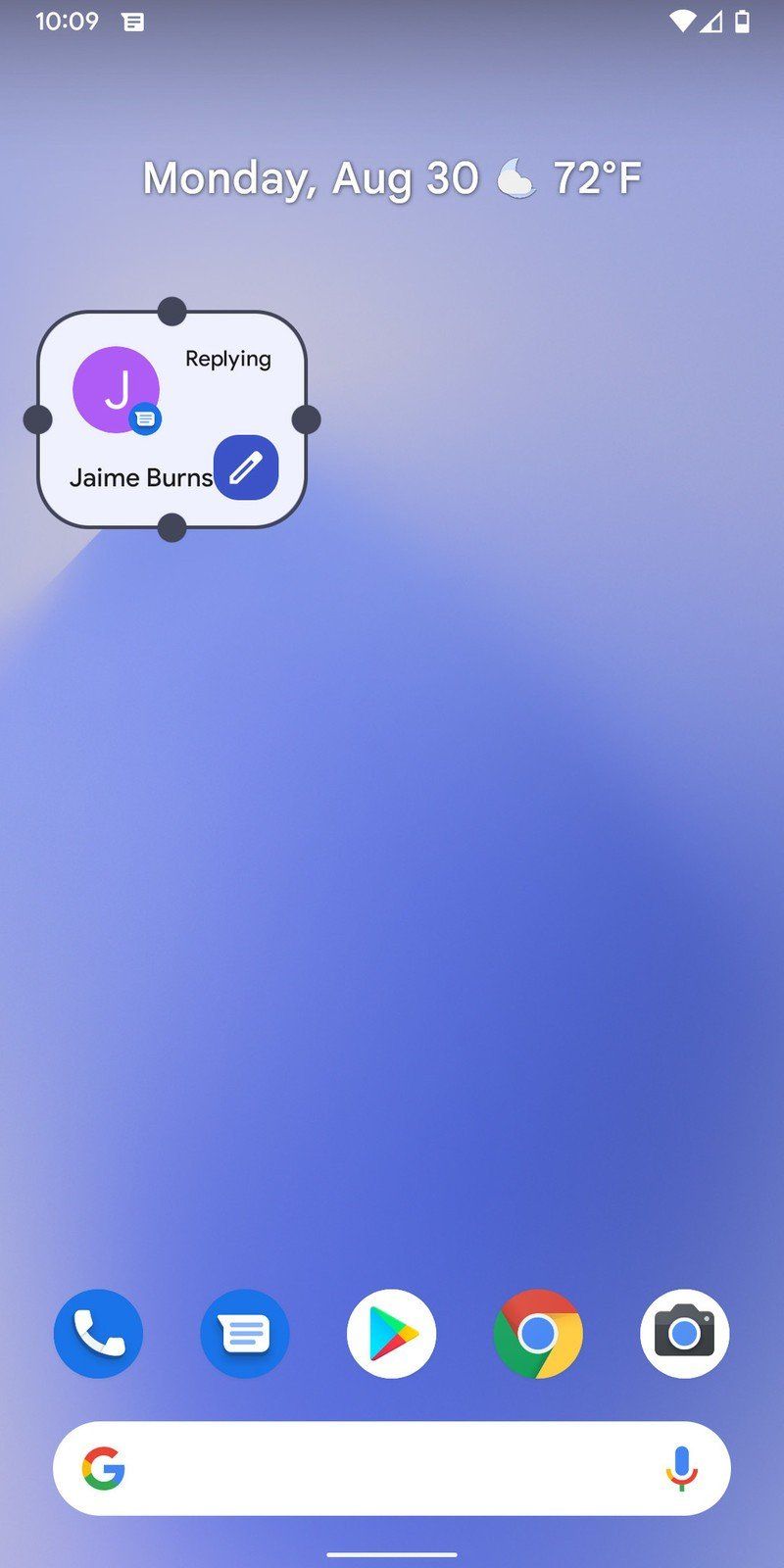The image displays the screen of a user's smartphone. At the very top left corner, in white text, the time is shown as "10:09." Adjacent to it on the right, there are two signal bars and a battery icon indicating about 50% charge remaining. 

Directly beneath this, spanning across the screen in white text, the date "Monday, August 30th" is visible. Accompanying the date, there is a crescent moon icon partly obscured by a cloud, symbolizing night time weather conditions, with a temperature displayed as "72°F."

Below this, on the left side of the screen, there is a small square with rounded corners, outlined in dark gray with a polka-dot pattern on each side. At the top of this box, black text reads "Replying." Inside the box, a white letter 'J' is centered within a filled purple circle, beneath which the name "Jamie Burns" is displayed. An edit button is also present within this square.

The content on the screen largely concludes here, except for the array of app icons situated at the bottom. From left to right, the icons are for the phone app, text messaging app, Google Drive, Chrome browser, and the camera app. Below this row of app icons is a white Google search bar, characterized by a multicolored capital 'G' on the left side and a vibrant blue and red microphone icon on the right.